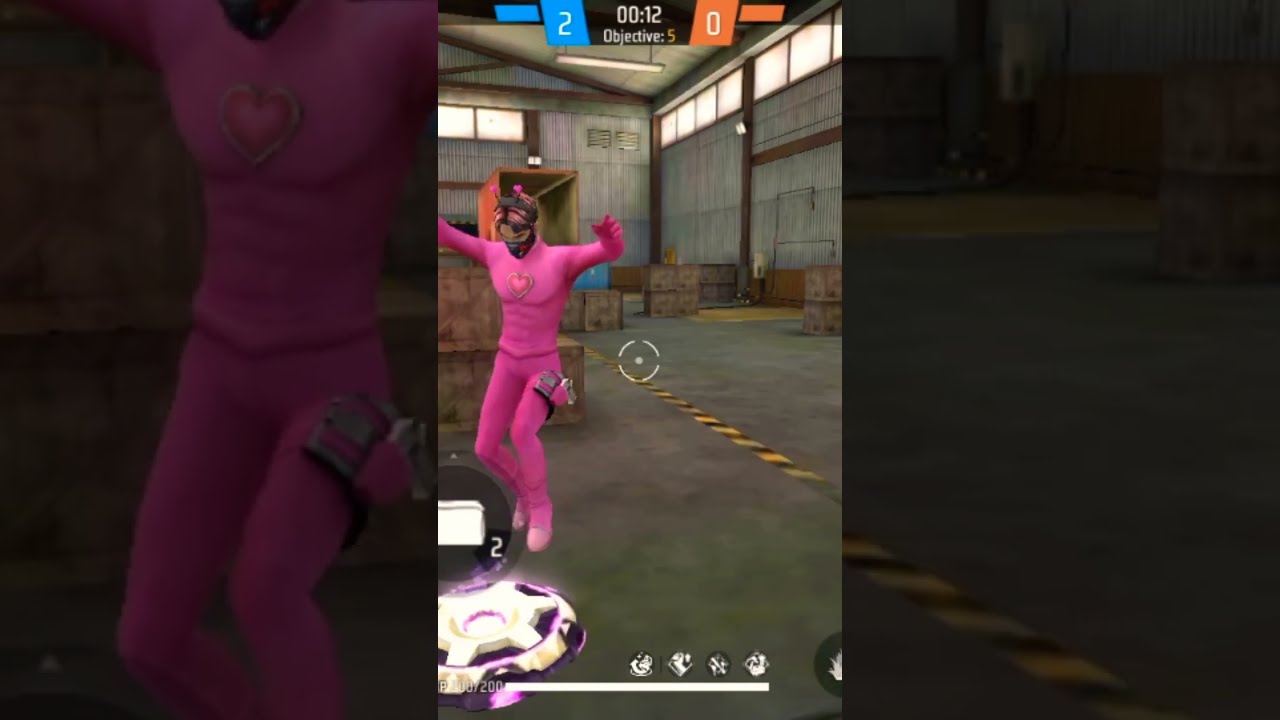This detailed screenshot captures a moment from a smartphone video game set in an industrial, warehouse-like environment. The top of the screen features two blue bars with white numbers, indicating a score of 2 for the blue team and 0 for the red team. A clock in the middle shows 12 seconds remaining, and the game objective is listed as "Objective: 5." The scene below takes place in a warehouse with stone floors, stone walls, and wooden beams supporting a high ceiling illuminated by light streaming through opaque windows. Scattered brown crates and a caution tape pattern on the floor hint at the industrial and possibly hazardous nature of the space.

Dominating the scene is a character in a tight-fitting pink bodysuit, complete with a gold heart emblem on the chest and a black mask with pink highlights. This figure, possibly a superhero, is in an energetic pose with arms outstretched, suggesting they are in the midst of dancing or jumping. They appear to be landing or interacting with a glowing white circular object tinged with purple and pink hues. Additionally, a progress bar and various game indicators, possibly representing health or abilities, are visible at the bottom of the screen, enhancing the immersive gameplay experience. The edges of the screenshot are blurred, focusing the viewer's attention on the dynamic action in the center.